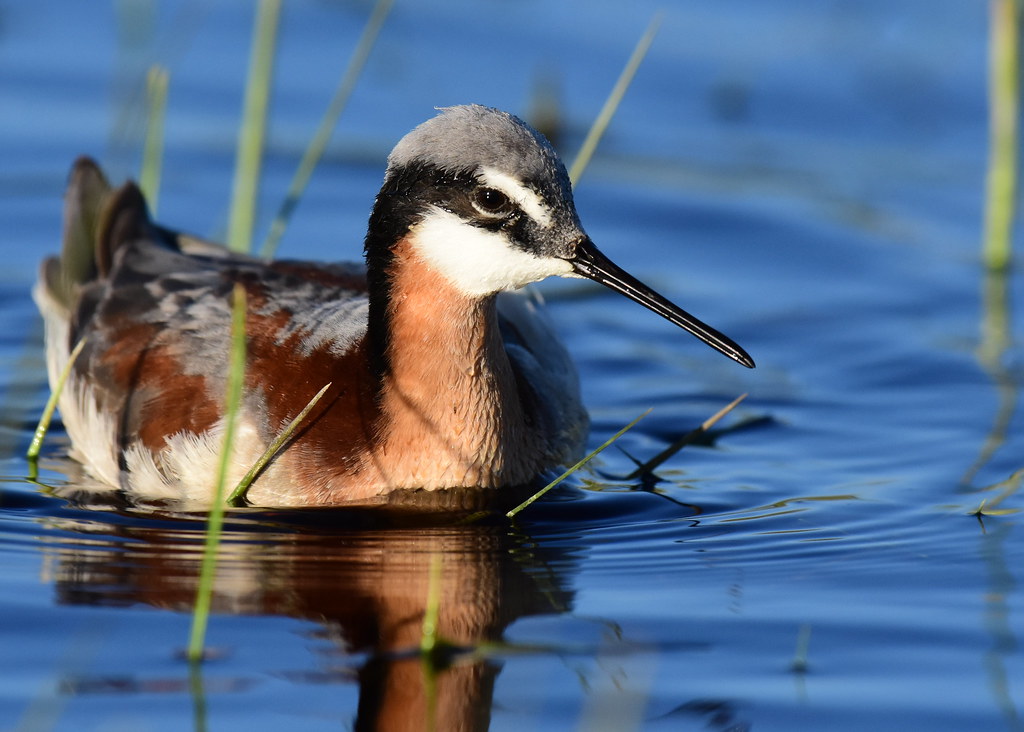In the foreground of the photograph, a bird floats serenely on a pond with occasional reeds emerging from the water. The bird, positioned centrally with its long, pointed black beak angled down and to the right, showcases a varied plumage. Its head is predominantly black, tapering into a grayish-pink hue atop, while the side of its head exhibits dark feathers with a distinct white patch above its eye. The neck features tan feathers on the front and transitions to a white underside beneath its chin. Its breast feathers are brown, and the back feathers appear reddish-brown in the light, with upright tail feathers completing the avian tableau. The bird's dark eyes project a sense of calm as it creates gentle ripples in the pond's reflective, bluish water. The overgrown reeds and foliage suggest a natural, tranquil pond setting. No text intrudes upon the scene, allowing the rich palette of browns, light browns, whites, blacks, grays, greens, and watery blues to fully convey the environment's peaceful atmosphere.